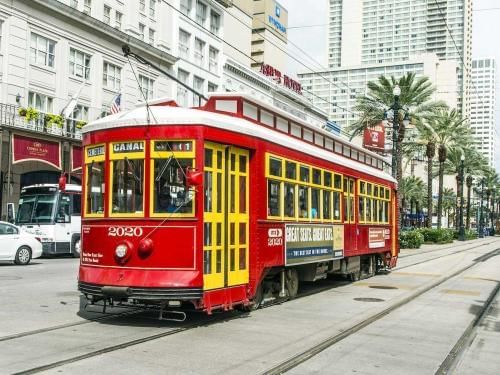The image depicts a realistic scene of a vibrant city street featuring a red trolley with yellow-trimmed windows. The trolley, marked with the number "2020" prominently displayed on its front, travels along its tracks down the middle of the road. There is an advertisement on its side that reads, "Great suits, great lots." Overhead, a cable connects the trolley to the tram line. 

Surrounding the trolley, there's a bustling urban environment with numerous palm trees—nine of which are clearly visible—lining the area between the tracks and the road. A variety of vehicles, including white cars and a bus, can be seen alongside the trolley. The background showcases an array of buildings, including very tall skyscrapers and multiple white apartment buildings, some with white pots filled with green plants bordering the street. 

Additionally, the image captures a nearby tram station, indicating the trolley is approaching a stop. Manhole covers punctuate the tracks, adding to the gritty detail of the cityscape. The scene is vivid and dynamic, exemplifying the lively nature of urban life.